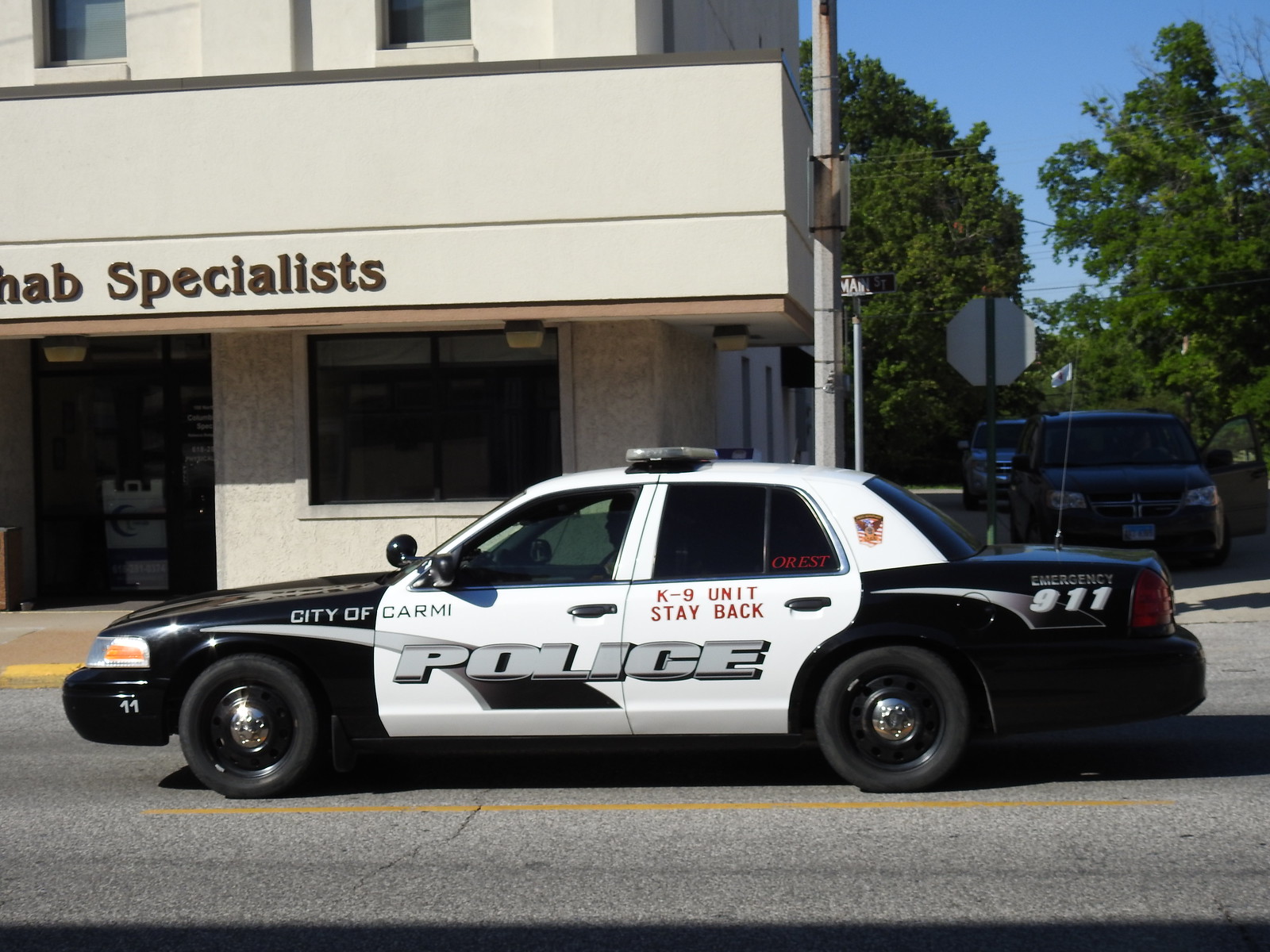A detailed photograph captures the side profile of a black and white police car, a four-door sedan with 'City of CARME, Police' inscribed in silver on its white body. The car features a black hood and trunk, and on its back door, red text that reads 'K-9, Unit, Stay Back' is clearly visible. The rear trunk also displays 'Emergency, 911' in silver. The rectangular-shaped light bar on the roof is currently off, appearing gray in the bright sunlight. The car is positioned on a gray asphalt road riddled with dark cracks, adjacent to a yellow lane divider. The vehicle, presumably in motion given the blurred details of its tires, is driven by an officer visible in the front seat. It appears to be halted near a beige building with black windows and doors, marked as a 'Rehab Specialist' facility. The building is lit by sunlight, and the clear, bright blue sky with no clouds suggests the photograph was taken on a sunny day, likely in spring or summer. The scene includes a backdrop of lush green trees and other parked cars along a cross street, indicating a tranquil, smaller city ambiance.